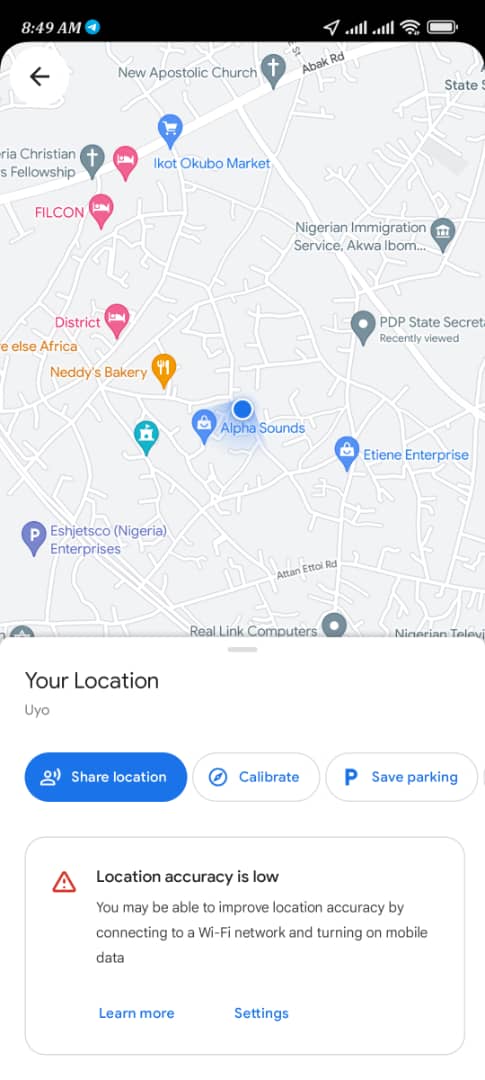A smartphone screen displays a detailed location map interface. At the top of the screen, encased in a black bar, the time reads 8:49 AM, alongside standard icons indicating full cellular signal, Wi-Fi connectivity, and a fully charged battery. Below this bar is a gray and white map dotted with various colored pins, including gray, blue, yellow, red, and green, signifying different points of interest.

In the upper left corner, the text "Your Location" is displayed in black. Directly below it, the location “UYO” is indicated. Beneath the map are several buttons: a blue "Share Location" button with white text, a white "Calibrate" button with blue text, and another white button labeled "Save Parking," also with blue text.

A notification at the bottom alerting the user of low location accuracy is present, suggesting that connecting to a Wi-Fi network and turning on mobile data may improve this. The notification is accompanied by a red triangle with an exclamation point, indicating urgency or an error. Additionally, options for "Learn More" and "Settings" are provided in blue text.

Various notable locations are marked on the map, including IKOTOKUBO Market, Philcon District, Nettie's Bakery, Alpha Sounds, and the Nigerian Immigration Services (aka WIBOM).

Overall, the screen provides a comprehensive map view with location-sharing capabilities and calibration options, while also offering guidance on improving location accuracy.